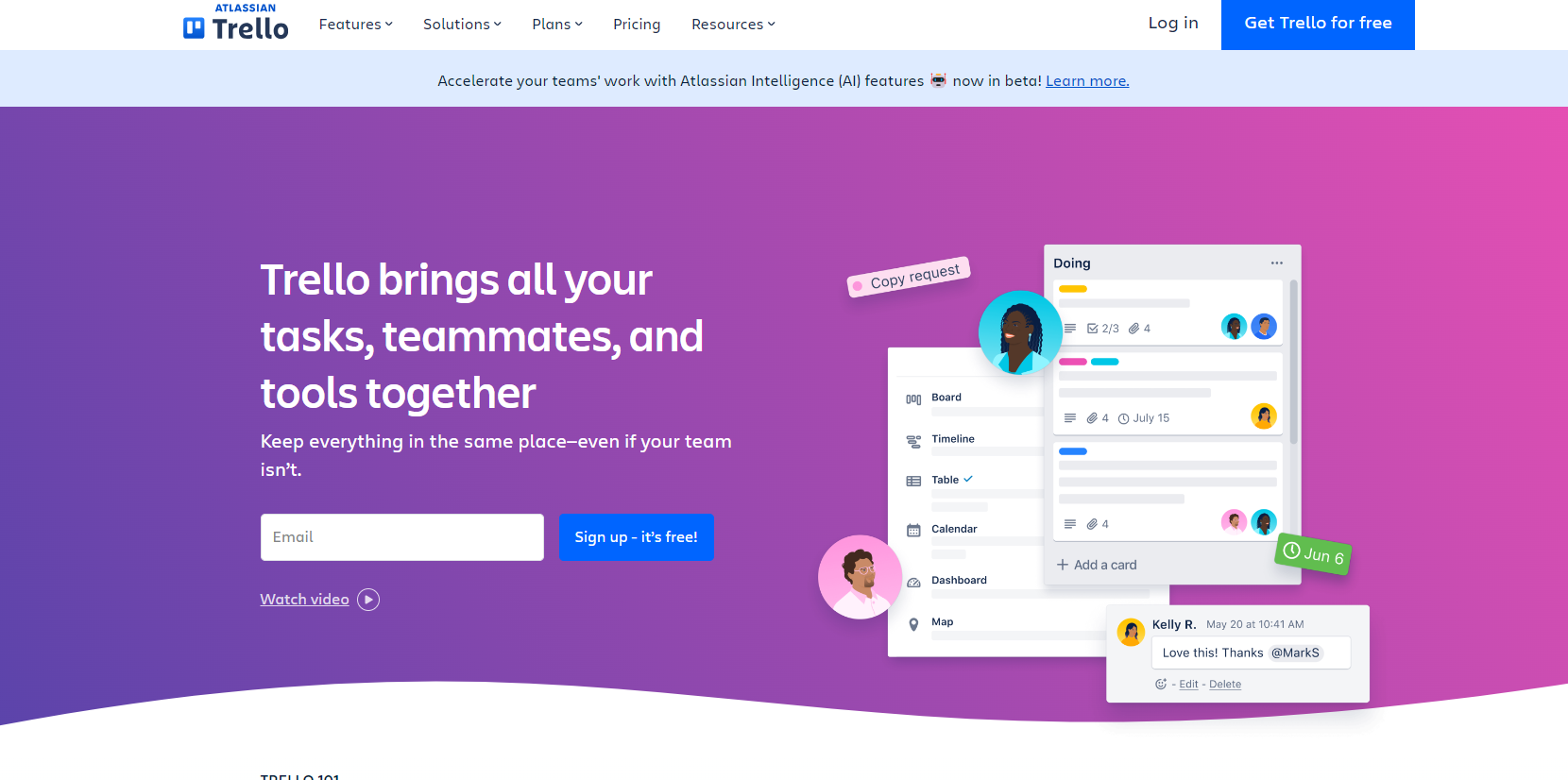The image showcases a segment of Trello's web interface with a predominately purple background at the top. On the left side, there's a small blue box with a 'P' inside next to the word 'Trello'. Directly below, a navigation menu displays options for Features, Solutions, Plans, Pricing, and Resources. On the right side of the header, there are buttons for "Log In" and a blue button that says "Get Trello for Free."

Beneath the top section, the purple background transitions into a light blue panel featuring a message in white text: "Accelerate your team's work with Atlassian Intelligence AI features." Accompanying this is a small, somewhat unclear icon with a 'Learn more' link.

Further down, the purple background resumes with a bold statement in white text: "Trello brings all your tasks, teammates, and tools together. Keep everything in the same place, even if your team isn't." Below this text are two buttons: a white button labeled 'Email' and a blue button labeled 'Sign up, it's free.' Close by, there is also a 'Watch Video' link.

To the right side of this section, there are some interactive elements, including a white flag labeled 'Copy Request' with a small red dot to its left. Additionally, there is an avatar of a young man within a pink circle, next to a blue circle containing a young woman's photograph. To the right of these avatars are two page icons accompanied by a small green box, and another small blue box with a yellow dot in its corner.